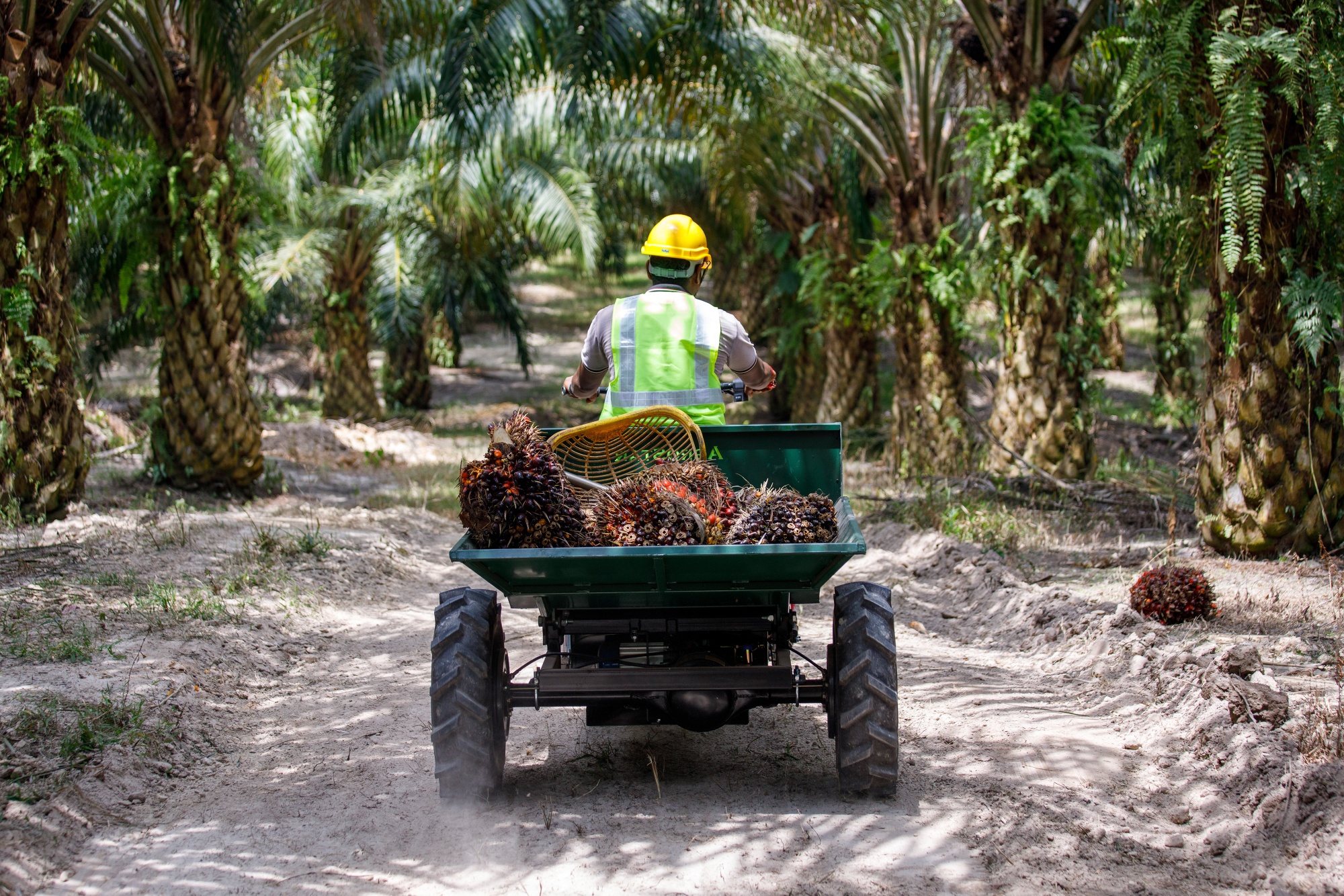In this horizontal rectangular photograph, a man is driving a small tractor through a forest of tall, unusual palm trees with large, spiky trunks and green fronds. The narrow, bumpy path beneath him is gray and sandy, dappled with shadows cast by sunlight filtering through the dense canopy. The driver, dressed in a green and gray reflective vest over a plaid shirt and wearing a yellow hard hat, navigates the rough terrain. The tractor's rear carry-all holds various pieces of fallen wood, tree roots, and large, spiky fruits. The scene is serene yet rugged, with the towering palms flanking the path and creating a partially enclosed, almost tunnel-like environment above.